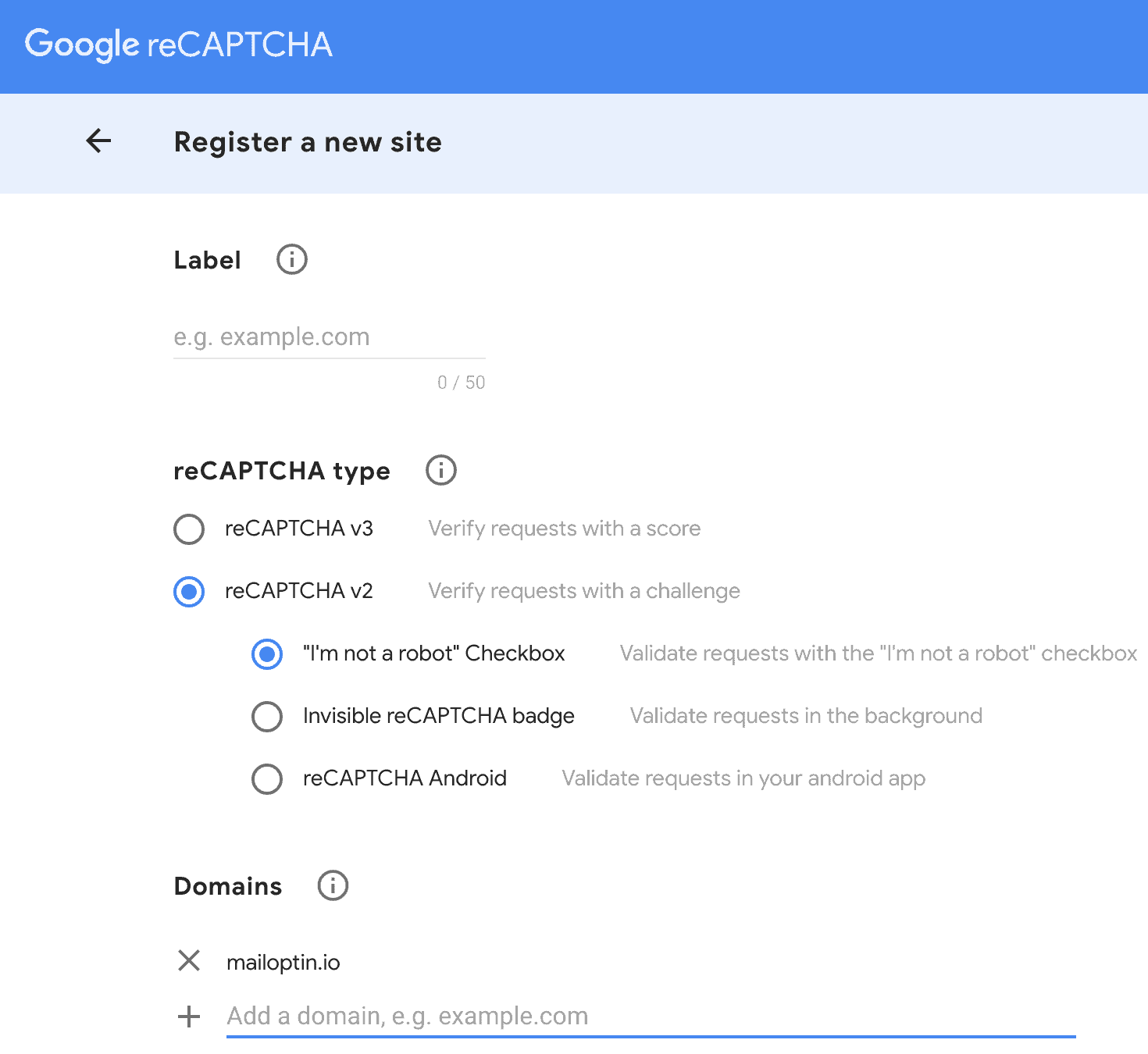The image displays a Google reCAPTCHA setup page with a refined and detailed layout. At the very top left, the "Google reCAPTCHA" logo is prominently displayed against a blue background with a white text stripe. Directly below, a gray-blue section labeled "Register a New Site" catches the eye, adorned with black text and an arrow pointing leftwards for navigation.

In the white background area underneath, the form to register a new site begins with a field titled "Label" accompanied by an informational button to provide additional context. The following input field suggests an example domain, "e.g., example.com," instructing users where to type their site name.

Further down, the section titled "reCAPTCHA Type" offers a selection of options, each with an informational button: 
- reCAPTCHA v2: Verify requests with a score
- reCAPTCHA v2: Verify requests with a challenge (the "I'm not a robot" checkbox)
- Invisible reCAPTCHA badge: Validate requests in the background
- reCAPTCHA Android: Validate requests in your Android app

Following this, the "Domains" field lists "mailoptin.io" with an 'x' button nearby, presumably to delete this domain. Users can also add new domains as needed, with the process supported by informational buttons to aid understanding.

Overall, the page is well-organized with clear sections and helpful tooltips, making it user-friendly for setting up Google reCAPTCHA on a new site.